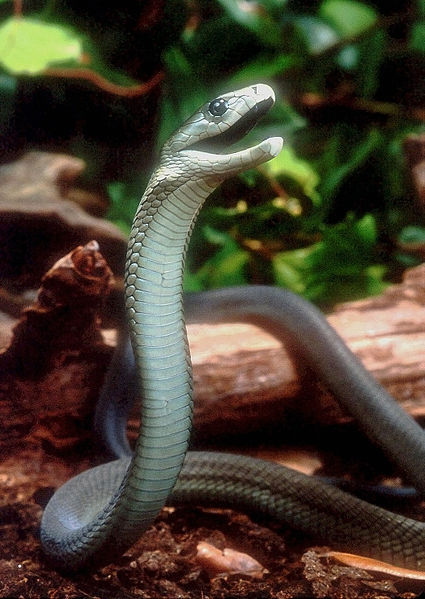The image is a highly detailed, outdoor close-up photograph of a greenish-gray snake, with a tan belly and scales meticulously depicted across its body. The snake, centered in the image, has its head lifted and neck extending downwards to the lower left, then curving back into the background and slightly reappearing in the lower right, suggesting a curled posture. The snake's open mouth reveals partially visible fangs and a single black eye on its right side. The background is blurred, featuring lush green foliage and a thick, broken, brown tree log behind which the snake partly coils. The ground in the foreground is brown soil, adding to the overall natural setting. Despite the realistic appearance, the cleanliness of the snake and surrounding elements hint that this photograph might have been captured within a controlled environment, such as an aquarium.